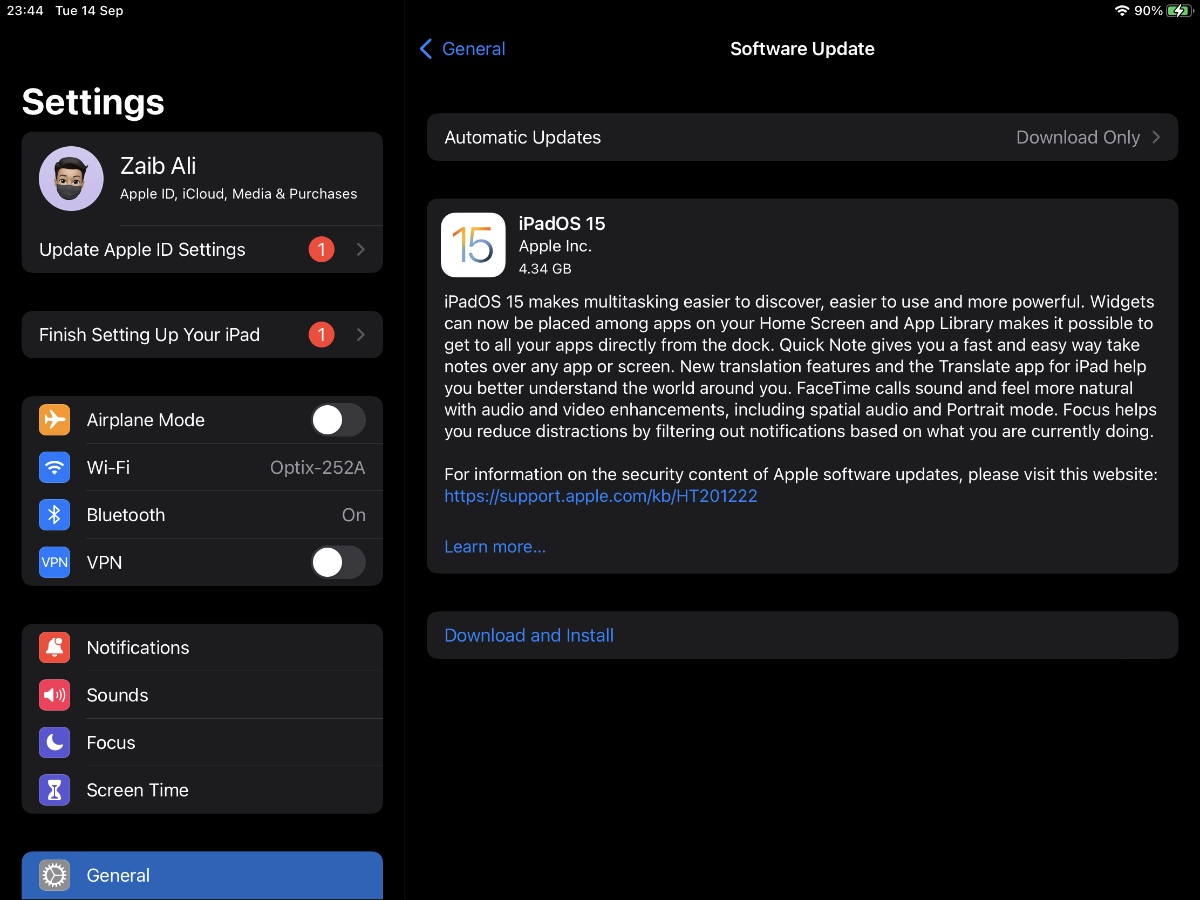This is a detailed screenshot of an iPad's settings app displayed on a computer screen, possibly emulating a mobile device due to the presence of battery and connectivity icons at the top. The battery indicator on the top right shows the device is currently charging and is at 90% capacity. The time displayed is 23:44, and the date is Tuesday, 14 September. 

At the top of the screen, the title "Settings" is visible, followed by "Zabe Ali, Apple ID, iCloud, Media & Purchases." Along the left sidebar, there is a series of icons and options, beginning with a prompt to "Update Apple ID Settings," indicated by a white exclamation mark in a red circle. This is followed by another alert to "Finish Setting Up Your iPad."

Below these alerts, eight icons are listed vertically with corresponding labels: Airplane Mode, Wi-Fi, Bluetooth, VPN, Notifications, Sounds, Focus, and Screen Time. Each option includes an associated icon for quick identification. At the bottom of the sidebar, the "General" settings option is highlighted.

To the right, details about an available software update for iPadOS are presented. Specifically, the update is titled "iPadOS 15" from Apple Incorporated and requires 4.34 GB of storage space. The section includes a paragraph explaining the update and offering options to "Download and Install."